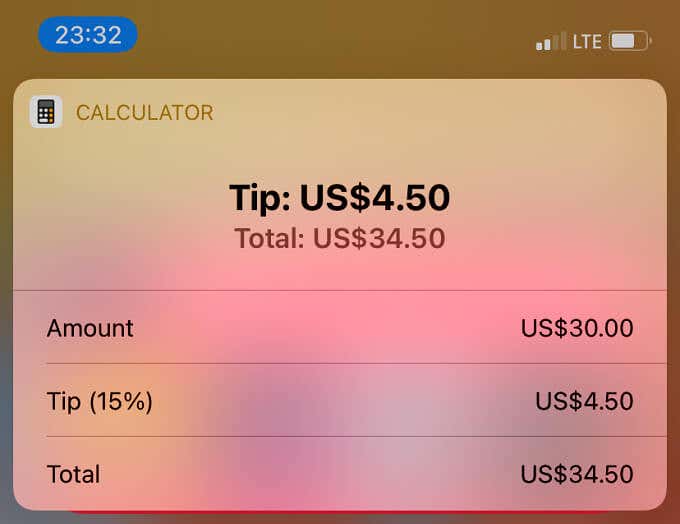This image showcases a tip calculator displayed on a smartphone screen. In the top left corner, the time is shown as 23:32 within a blue capsule, while to the right, the network signal indicates two out of four bars next to an LTE symbol and a battery icon approximately 60-70% charged. The blurred background appears brownish, with an upper overlay field in a pink or beige hue, displaying further blurred colors possibly from an image beneath.

Central to the image is an application interface marked by a calculator icon in the upper left and the title "Calculator." The main feature includes fields labeled "Tip" and "Total." The word "Tip" is prominently displayed in large black text, while "Total" appears below it in maroon or purple text of a slightly smaller size. The calculator details are as follows:

- **Tip:** USD $4.50
- **Total:** USD $34.50

Below are three lines providing a breakdown:
- **Amount:** USD $30.00
- **Tip at 15%:** USD $4.50
- **Total:** USD $34.50

This user-friendly tip calculator app is intended to assist patrons in quickly calculating gratuity, especially useful in restaurant settings when mental math might be challenging, such as after consuming a few drinks. This ensures correct tipping, facilitating a seamless dining experience where everyone is content.